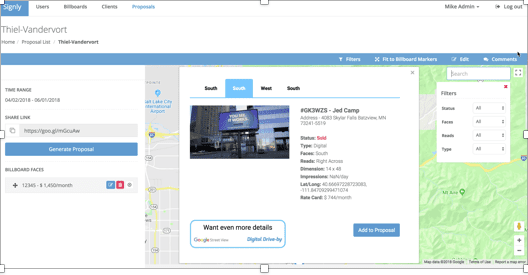This image is a small screenshot of the upper left corner of a web page with a white background. In the upper left corner, there's a blue square with the word "Signally" in white font. To the right of this square, there are navigation links labeled "Users," "Billboards," and "Clients and Proposals," with "Proposals" highlighted in blue. In the top right corner, the text "Mike Admin" is displayed next to a "Log Out" button.

Below this, there's a white rectangle featuring the text "Thiel-Vandervoort" in black font. Underneath, a breadcrumb navigation reads "Home / Prog Out List / Thiel-Vandervoort," though it is somewhat difficult to read. Additional text below this indicates a time range: "04/02/2018 - 06/???" with the latter part illegible. 

Further down, the phrase "Share Link" appears in black font, followed by a gray field containing a URL: "https://GU/GI certificate."